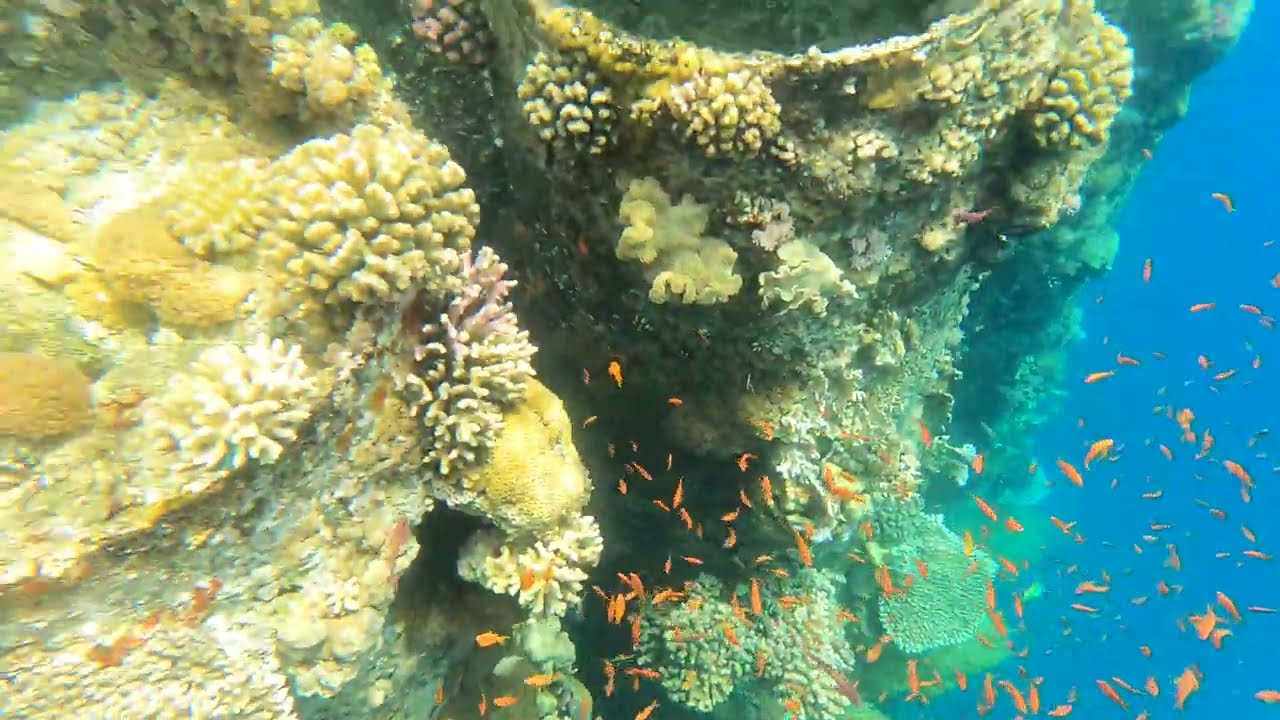This rectangular underwater image, approximately 8 inches wide by 4 inches tall, vividly captures a bustling coral reef scene. Dominating the composition is a coral structure teeming with diverse coral types, including starburst-shaped formations and curly, lettuce-like growths in shades of yellow, beige, and dull green. Some corals resemble flowers, while a patch of it shows signs of bleaching or decay. An intriguing detail suggests that the reef may have developed around a sunken, artificial structure, providing a unique and striking visual. Hundreds of tiny, vibrant orange fish, reminiscent of goldfish, swim around the coral in a large school, adding life and motion to the scene. The water surrounding this underwater community is a deep, vivid blue, enhancing the striking contrast and clarity of the image.